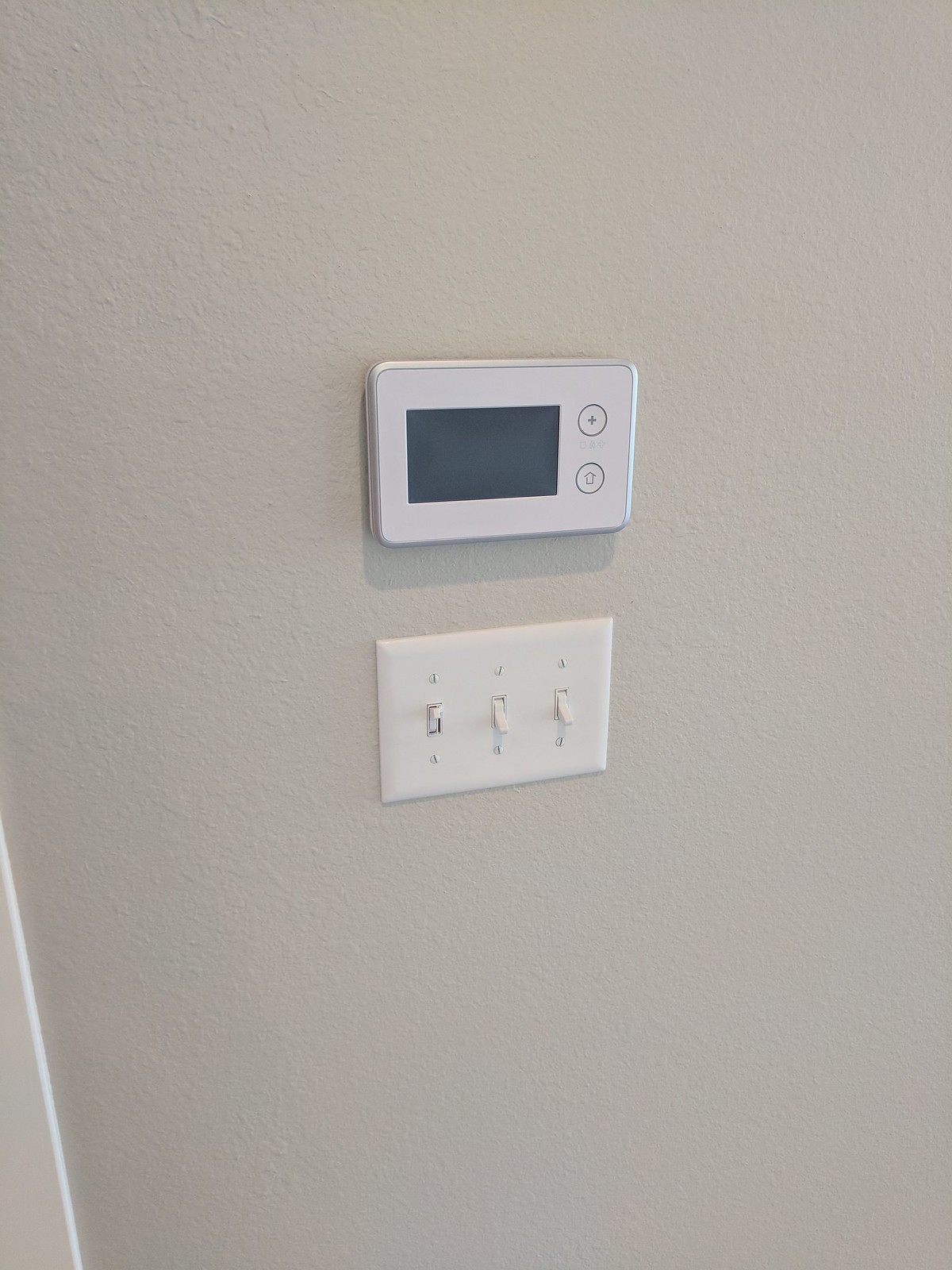The image showcases a section of a beige-gray wall inside a house. In the center of the wall is a white programmable thermostat featuring a black touchscreen. Adjacent to the touchscreen is a plus sign, and beneath it is an arrow button for additional controls. Directly below the thermostat is a light switch panel consisting of three individual switches. The left-most switch is turned on, while the middle and right switches are off. Each switch is secured by screws positioned above and below. The wall itself lacks any additional decorations, but the lower left-hand corner reveals a piece of white trim. The surface of the wall has a subtle texture, contributing to its soft, grayish-tan hue. The overall scene is minimalistic and unembellished, with no active display on the thermostat and only a single light switch engaged.